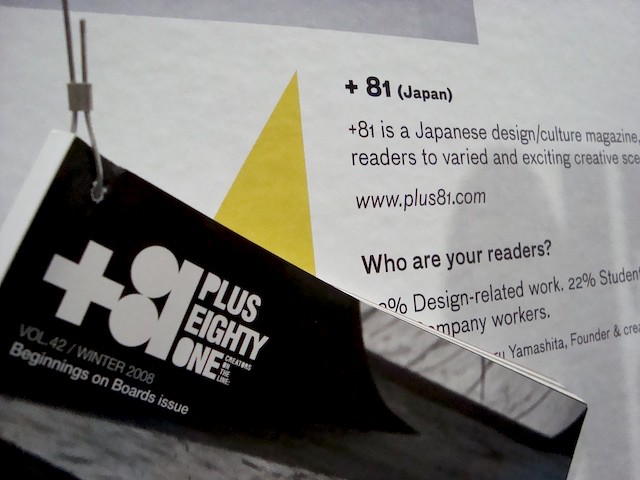The photograph captures a close-up view of a white wall adorned with black text and geometric shapes, including a large gray square and a yellow triangle. Prominently displayed on the wall is a description of "+81 Japan," identified as a Japanese design and culture magazine. Though some of the words are cut off, the legible text reads, "Plus81 Japan. Plus81 is a Japanese design culture magazine. You can read it to a varied and exciting creative scene. www.plus81.com. Who are your readers? Design related work, 22% student workers, Yamashita, founder and creator."

Hanging from the wall, attached by a silver wire, is a small black booklet titled "Plus 81, Creators on the Line, Volume 42, Winter 2008, Beginnings on Board Issue." This booklet and the precise, organized layout of the wall create an intriguing visual, merging elements of graphic design with physical media.